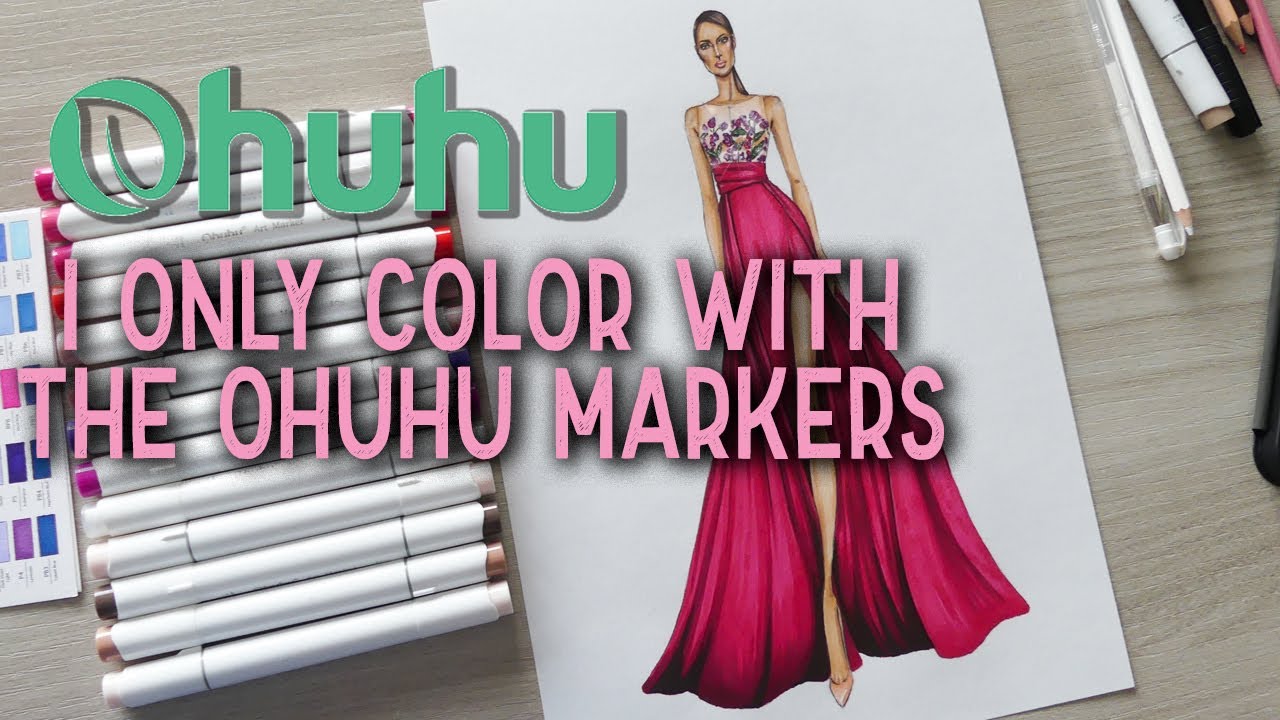This indoor photograph captures a detailed illustration on white paper, set on a wooden table. The central focus is a drawing of a tall, elegant white woman with dark brown hair in a ponytail, dressed in an eye-catching outfit. The lower half of her dress, a long red garment, flows down to the floor, with a split revealing one of her legs. The top part of her dress features a floral print with white and purple flowers, adding a delicate touch to her attire. She appears serene and unsmiling. Surrounding the drawing, the table holds a collection of white Ohuhu markers with colorful caps arranged on the left side, and a few pencils and pens placed diagonally on the right. Additionally, there's a notable green logo featuring a leaf outline at the top left of the paper, beside the text, "Ohuhu." Below this in pink, it's written, "I only color with the Ohuhu markers." The image captures the artistic tools and drawing within a neatly organized, creative setup.